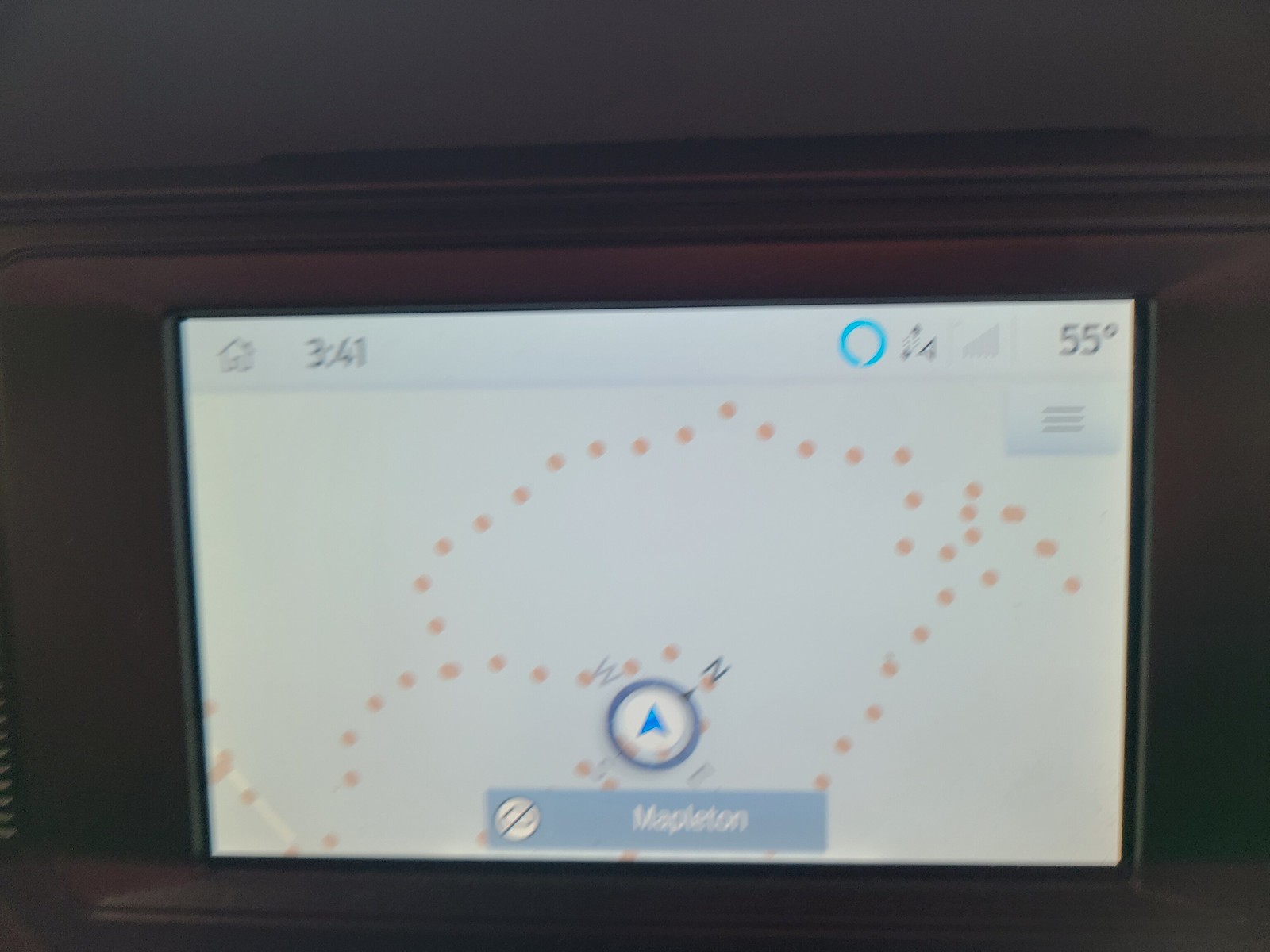The image depicts a close-up of an LCD display, possibly from a car dashboard, against a dark brown background. The top left corner of the screen features a home icon followed by the digits "341." Adjacent to this on the upper right, a bright blue circle displays the temperature "55 degrees." Below, at the center bottom, a blue rectangle with white text reads "Mapleton" (M-A-P-L-E-T-O-N). Above this rectangle, a navigation map is shown with a blue arrow in a white circle, surrounded by a compass indicating directions (north, east, west, south) and dotted with multiple beige or light orange dots, which may represent the area or a footpath. The display also includes a faint light paneling strip, further adding to its intricate design.